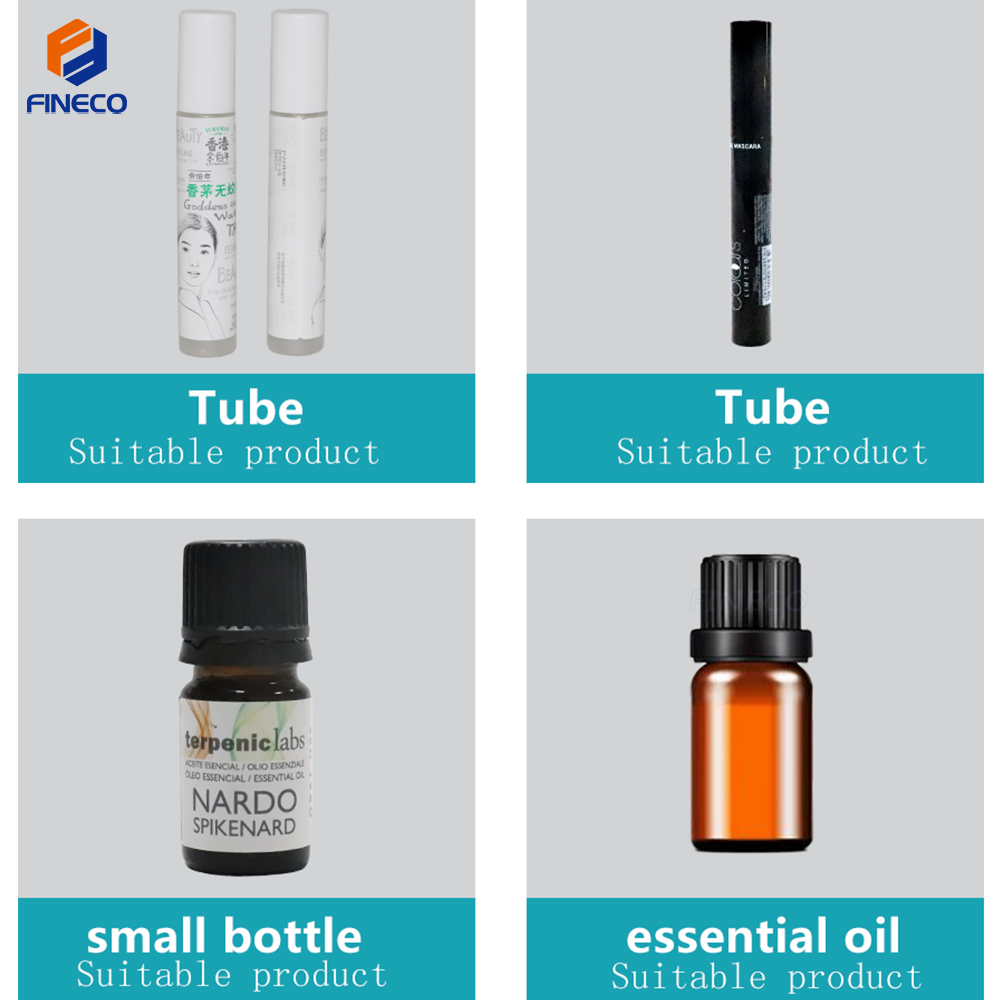The image is a squared collage consisting of four product photos, each separated by a thick white border and set against a gray background. In the top left-hand corner of the image is the Fineco logo, which features an orange "F" intertwined with a blue "F" rotated 180 degrees, with "Fineco" written in blue text below it. Each product photo has a rectangular teal box at the bottom, with large white text indicating the type of product: "Tube," "Small Bottle," or "Essential Oil," followed by the phrase "Suitable Product."

- **Top Left Photo:** Features a white tube with Chinese text on it. Beneath this image, within the teal box, it says "Tube, Suitable Product."
- **Top Right Photo:** Displays a black tube, similar in appearance to a mascara container. The teal box also reads "Tube, Suitable Product."
- **Bottom Left Photo:** Shows a small glass vial with a white label. The label reads "Trepanic Labs Nardo Spike Nard," and the teal box underneath says "Small Bottle, Suitable Product."
- **Bottom Right Photo:** Depicts a small amber glass bottle with a black twist top, labeled as an essential oil. The teal box below it says "Essential Oil, Suitable Product."

The combination of these details emphasizes the cohesive presentation and branding of Fineco's products within the collage format.